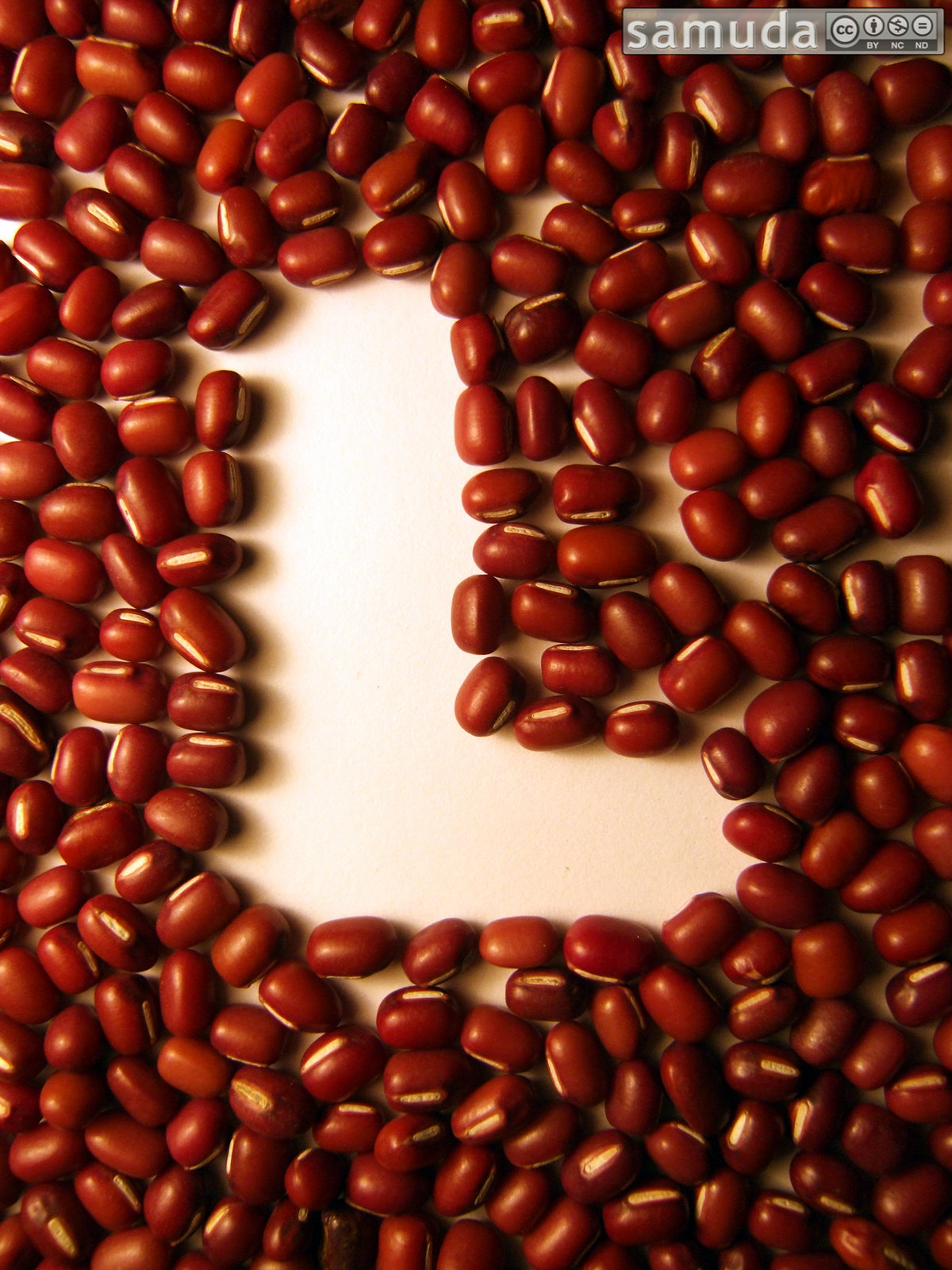This color photograph, titled "Samuda," prominently features numerous brown beans arranged on a slightly off-white surface. At the top right corner of the image, the name "Samuda" is visible, accompanied by additional, smaller graphics or text. The beans, which could potentially be kidney beans or even light coffee beans, are dispersed across the background and purposefully positioned to form the letter "L" in the center. The careful spacing and arrangement of the beans against the stark, clean backdrop accentuate the intended shape, creating a simple yet visually striking composition.